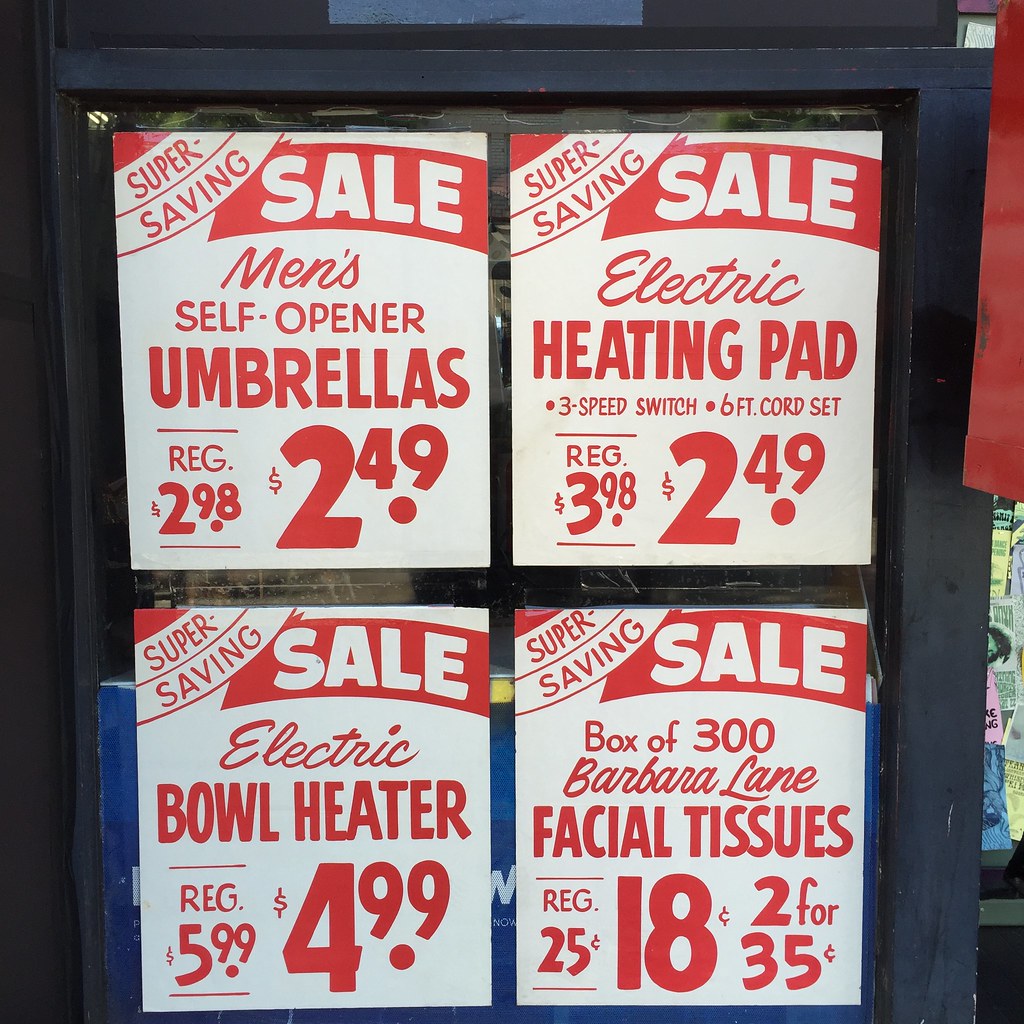The image depicts a store window display featuring four prominent sale flyers, all with a consistent white background and red lettering, framed by a black border. Each flyer is part of a "Super Saving Sale" promotion, with the words "Super Saving" in a white border with red letters, and "Sale" in a red border with white letters. 

- The top left flyer advertises Men's Self-Opening Umbrellas, regularly priced at $2.98, now available for $2.49.
- The top right flyer promotes an Electric Heating Pad with a three-speed switch and a six-foot cord, marked down from $3.98 to $2.49.
- The bottom left flyer features an Electric Bowl Heater, reduced from $5.99 to $4.99.
- The bottom right flyer offers a Box of 300 Barber Lane Facial Tissues, originally $0.25, now $0.18 or two for $0.35.

In the background, various grocery items in colorful boxes, primarily yellow and blue, are visible on the right side, while the left side remains dark with a piece of blue tape at the top of the board.